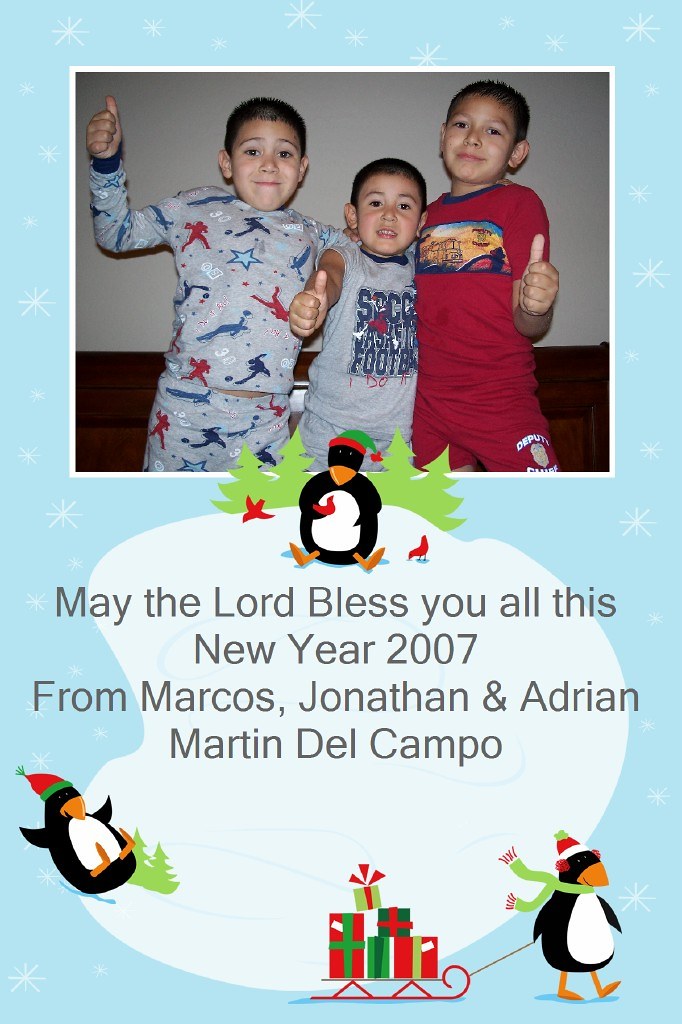The holiday Christmas card is a tall, rectangular digital image with a light sky-blue background adorned with tiny white snowflakes. At the top half of the card, there's a wide rectangular photograph framed with a thick white border, featuring three young boys who appear to be Hispanic, all smiling and giving a thumbs up. The boys stand in front of an off-white wall and a dark brown bed frame. 

The boy on the left is dressed in gray pajamas adorned with blue, dark blue, and red action figures, while the boy in the middle wears a gray shirt with blue text that says "soccer" and "football." The boy on the right is in dark red pajamas with a logo at the center. All three boys have tan skin and short black hair. 

Below the photograph, there is an illustration of three playful penguins. The central penguin sits wearing a green and red Santa hat, surrounded by green trees in the background. To the bottom left, a penguin with a red and green hat slides down, while the bottom right features a penguin in a green scarf and red-and-white elf hat, pulling a red sleigh filled with presents in various red and green colors. 

In the space between the penguins, the text reads: "May the Lord bless you all this New Year 2007 from Marcos, Jonathan, and Adrian Martin Del Campo" in gray font on a white piece of snow.